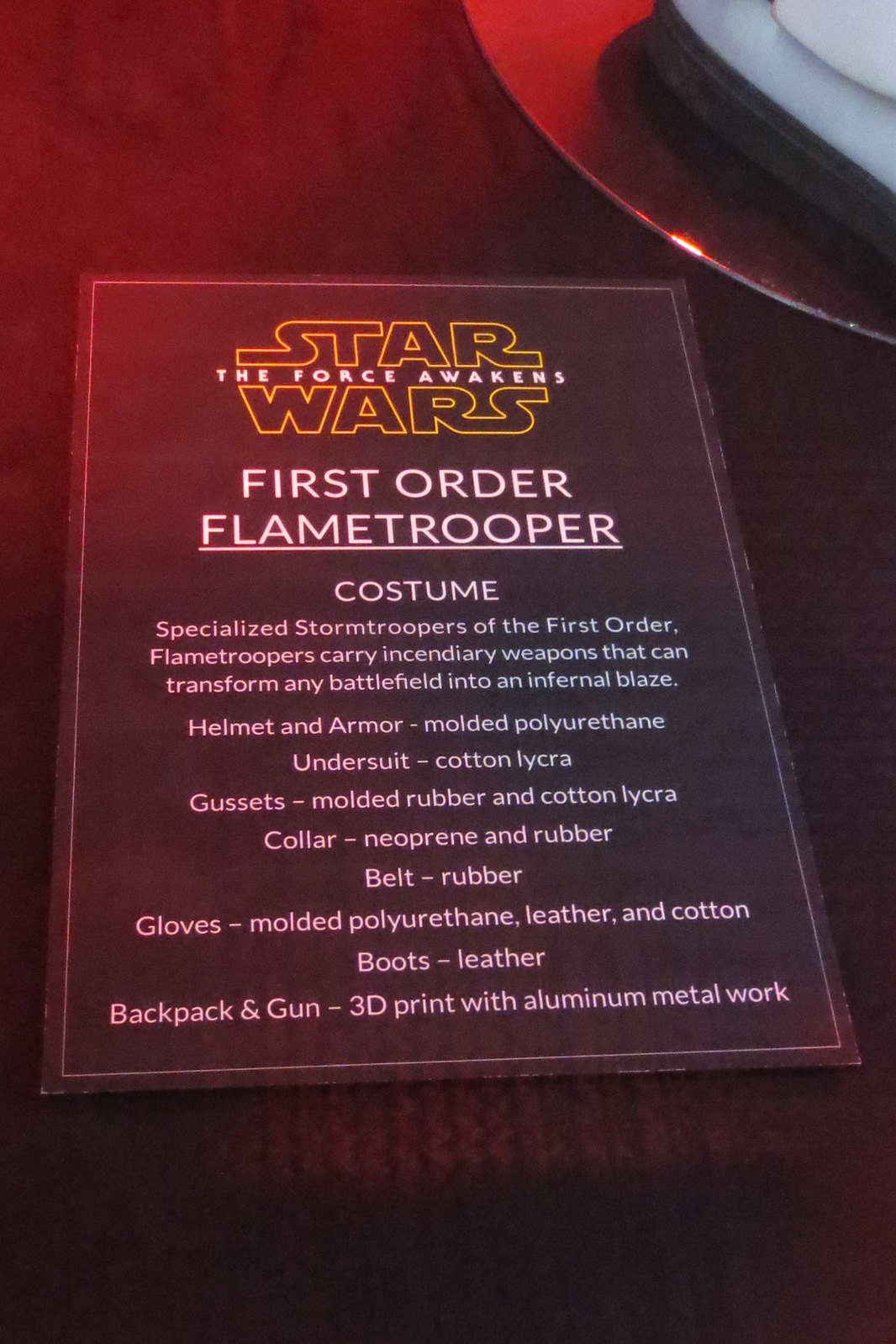This photograph captures a richly detailed scene set at the edge of a redwood dinner table. At the upper right corner of the table, a burgundy-colored plate, harmonizing with the table’s hue, holds what appears to be a neatly folded napkin. Dominantly resting on the table is a black pamphlet bordered in orange, closely matching the table's color tones.

The pamphlet prominently features the Star Wars logo at the top, with the text "The Force Awakens" nestled in between the words "Star Wars," which are displayed in large, yellow-outlined, black uppercase letters. Below this, in white uppercase letters, the pamphlet reads "First Order Flame Trooper" on two lines. Beneath this, the word "Costume" is written in smaller white text.

The pamphlet provides intricate details about the Flame Trooper costume, including that these specialized Stormtroopers of the First Order carry incendiary weapons capable of transforming any battlefield into an immense blaze. The description details the materials used for various costume components: helmet and armor made of molded polyurethane; undersuit of cotton lycra; gussets of molded rubber and cotton lycra; collar of neoprene and rubber; belt of rubber; gloves of molded polyurethane, leather, and cotton; boots of leather; and the backpack and gun, which are 3D-printed with aluminum metalwork.

In addition, a gold plate shimmers subtly in the background, contributing to the cohesive and well-balanced composition of the scene.